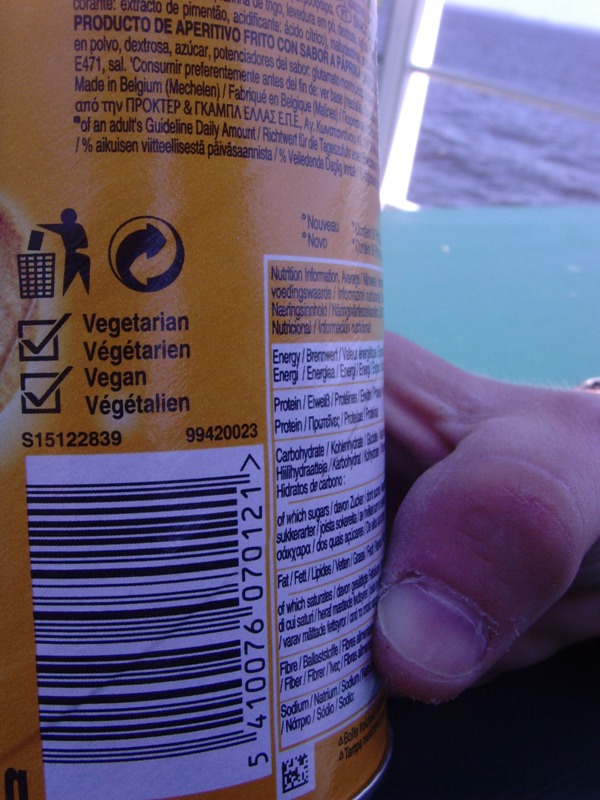In the image, a person's right hand is seen holding an orange-colored can prominently labeled with "vegetarian" in multiple languages — English, French ("végétarien"), and possibly Spanish or Italian. The can also features a "vegan" label, and all the vegetarian checkboxes are marked. Additionally, there is an icon of a man recycling a can, indicating the product’s eco-friendly packaging. A scannable barcode is visible along with some nutrition information, which is partially legible and suggests that the product might be an energy drink. The setting seems to be on a boat, inferred from the blue table in the foreground and a window behind, revealing an expansive view of the ocean. The person's thumb is wrapped around the right side of the can, obscuring the rest of their fingers. The image captures the serene maritime environment and the commitment to sustainable, vegetarian-friendly products.